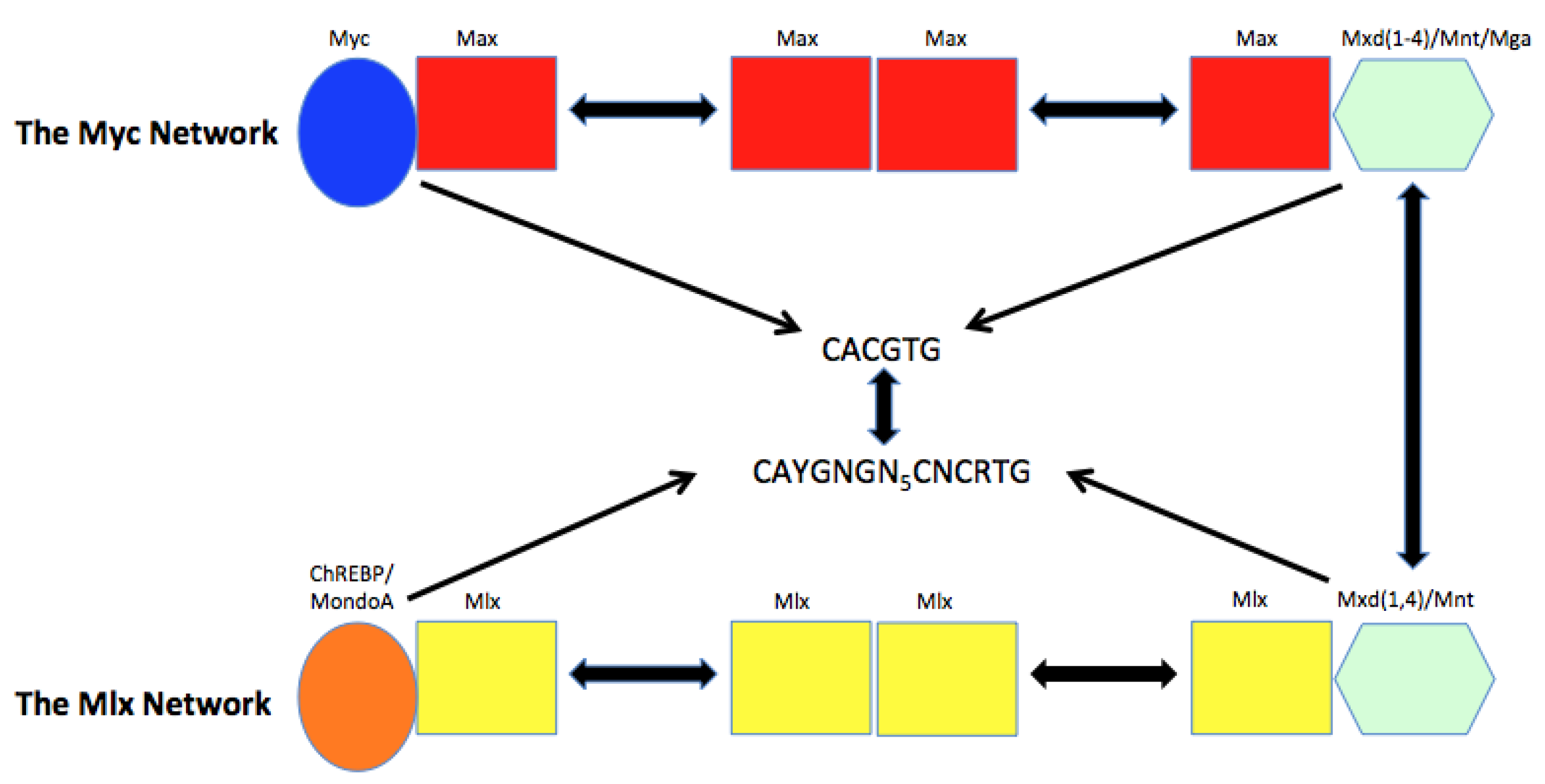The diagram features a detailed flowchart centralizing around the acronym "CACGTG." This central panel is interconnected by black arrows pointing up and down to a double-sided arrow that bridges "CACGTG" with "CAYGNGN" and "CNCRTG." Surrounding this core text, the image is populated with consistent shapes and labels across four quadrants, all converging towards the center.

In the upper left corner, there is a blue oval labeled "the MYC Network," flanked by several red squares bearing black arrows, some labeled "MAX." These arrows flow between the shapes in a multi-directional pattern. In the lower left, an orange oval labeled "the MLX Network" is present. This quadrant also includes four yellow squares separated by two black arrows.

On the right side of the diagram, the upper right corner shows a pastel green hexagon, which connects to a similar shape at the bottom with black arrows indicating directionality. Below, the formation mirrors the opposition with an orange oval labeled "mix network," along with green octagons labeled "MXD, 1-4, MMT, MGA."

The uniformity of the top and bottom rows is underscored by repetitions of blue circles, red squares, and pastel green hexagons/green squares. Detailed labeling of each shape appears above them, reinforcing the structured interrelation encapsulated by directional arrows from all corners towards the central text, outlining the intricate connections within the flowchart.